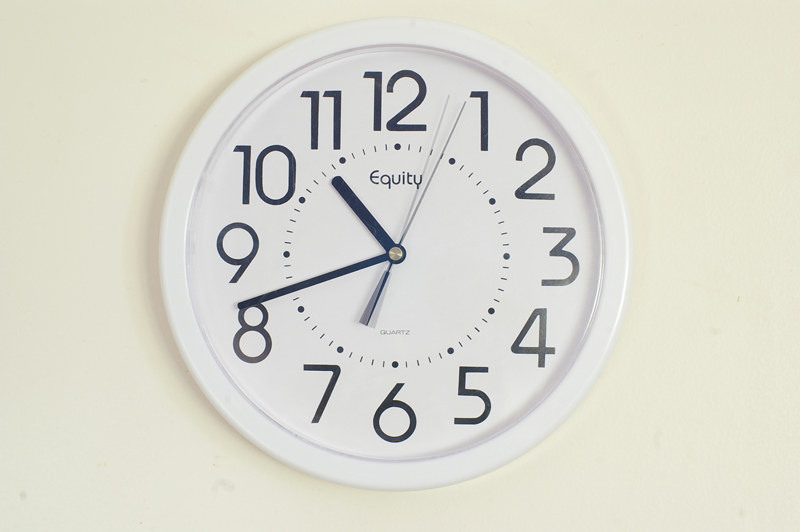The image features a plain white wall clock with a white frame and a white background, prominently displaying black numbers and hands. The clock is mounted on a light beige wall, which subtly contrasts with the white frame. Positioned in the center of the clock, the numbers are arranged in a standard format with 12 at the top, 6 at the bottom, 3 to the right, and 9 to the left. The clock has three distinct black hands: the longest and thinnest is the second hand, the medium-sized one is the minute hand, and the shortest is the hour hand. At the top center of the clock face, the word "Equity" is visible, with "Quartz" written in smaller text below it. Sunlight is softly illuminating the scene from the right, giving a clean, minimalist aesthetic suitable for a product listing on a website.